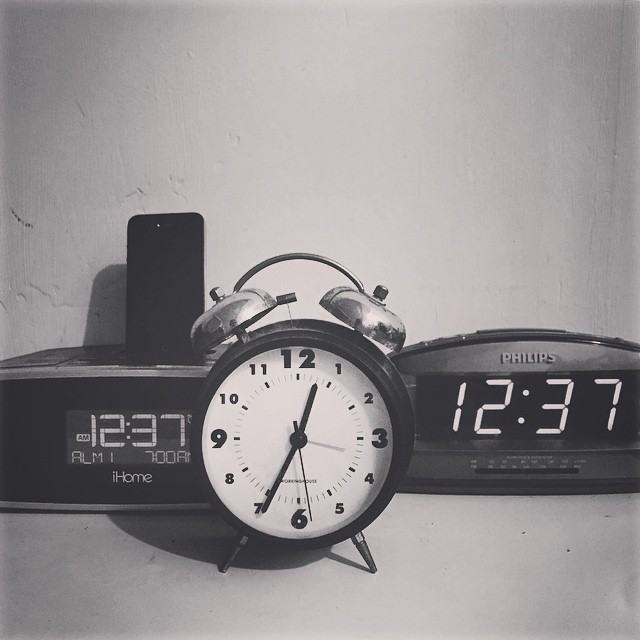This black-and-white photograph showcases three alarm clocks, highlighting the evolution of timekeeping devices across different eras. On the left, a modern iHome alarm clock made of black plastic is digitally displaying 12:37. It features a slot on top where an iPhone or iPod is vertically docked, indicating its capability to charge and play music. In the center sits a vintage-looking round analog alarm clock, characterized by its classic twin silver bells connected by an arch on top, which manually ring when the alarm sounds. To the right, a Philips digital alarm clock, reminiscent of designs from the 1990s or early 2000s, also shows the time as 12:37. The white wall and surface enhance the nostalgic feel of the image, creating a striking contrast with the modern elements, thus portraying the progression in alarm clock technology.